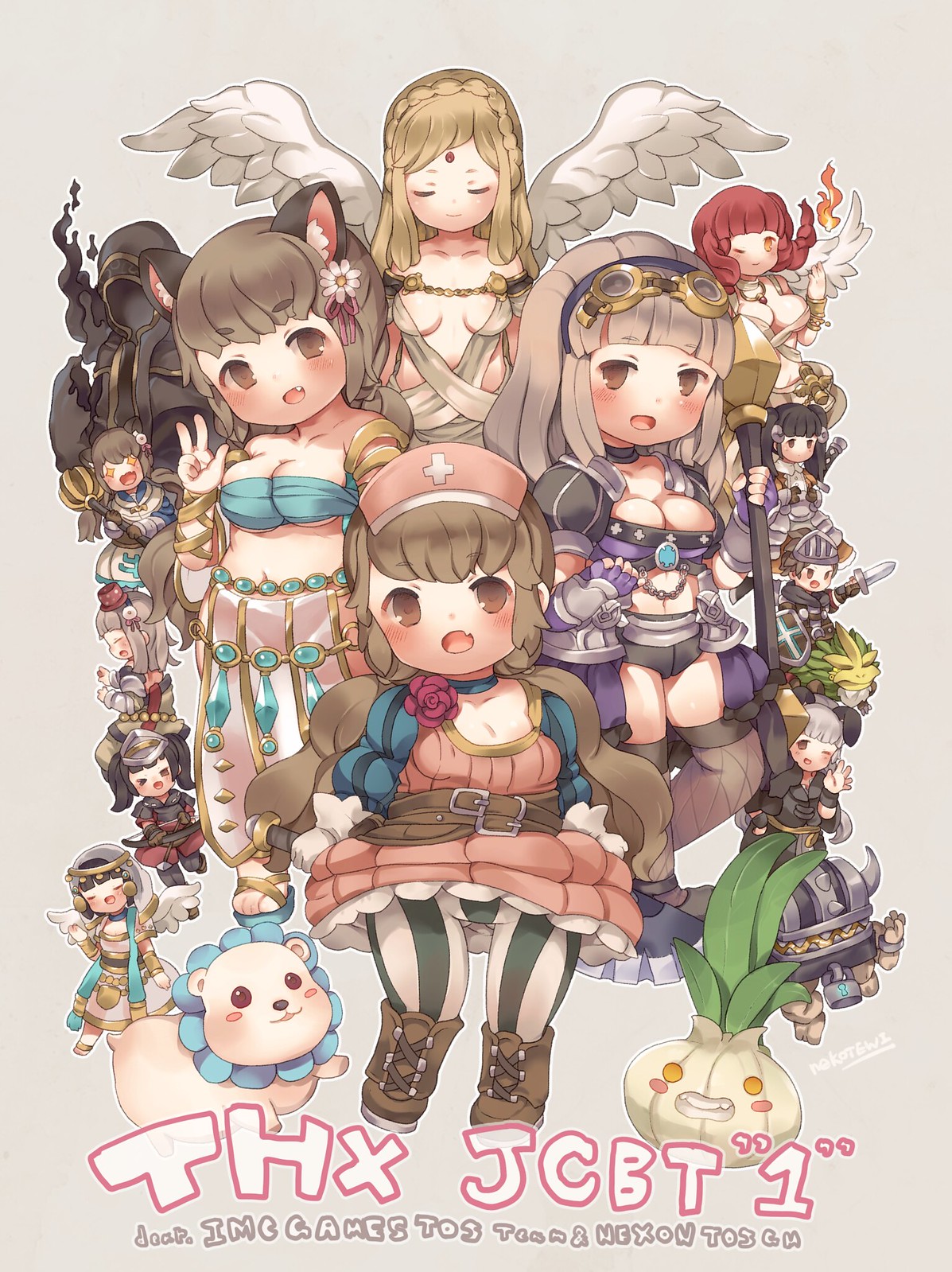This vibrant color illustration, created digitally or with watercolor and ink techniques, showcases a fantastical, anime-inspired scene filled with pastel hues that encompass the rainbow. At the center stands a group of four distinct anime characters with intricate, jewel-adorned outfits featuring belts. The central figure at the back is a young anime girl with angel wings, her head slightly tilted forward and eyes closed, adorned with a redstone on her forehead. Flanking her are two characters: on the left, a young girl with short brunette hair styled like cat ears, wearing a halter top and a leather skirt, looking into the camera; on the right, another with goggles on her head, dressed in a halter top and black shorts. In the foreground, an anime girl in a nurse’s uniform, complete with a hat and skirt, gazes directly ahead. The central three girls, slightly sexualized with blush on their cheeks and slightly open mouths, all have a small tooth visible and are staring straight at the viewer.

Surrounding the main group are several smaller floating figures, including a unique hooded character to the top left and additional women. Notably, a chibi lion can be seen in the bottom left, while an anthropomorphic onion with a face appears to the right of the central foreground girl. Besides these, the illustration includes various other smaller characters adding to the scene's depth. At the bottom, crafted in white text with a pink border, the text "THX JCBT1 (IMC Games)" is prominently displayed.